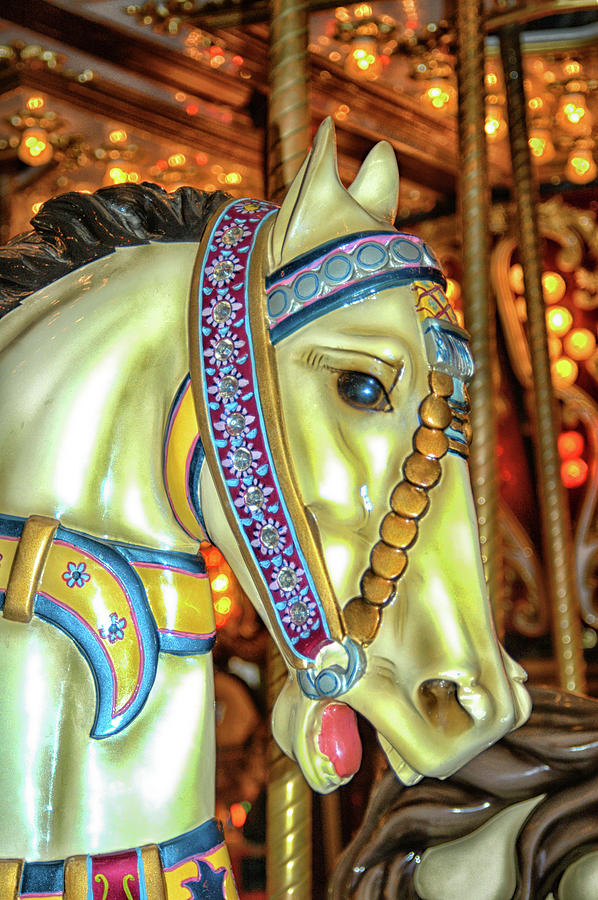The image features a vibrantly decorated horse on a classic carousel, bathed in a colorful and nostalgic ambiance. The horse is primarily white but adorned with a striking array of embellishments. Its face, turned to the right, displays a lively expression with flared nostrils, a bright pink tongue partially visible, and a haunting dark blue glass eye gazing at the viewer. A beautifully ornate bridle in magenta, adorned with blue and pink floral patterns, enhances its face, while a blue headband with gray circles adds a regal touch. The mane is meticulously detailed, and beads cascade down its face.

The horse's body is dressed with a yellow ribbon bordered in blue around its neck, and it is anchored to the carousel by the iconic golden pole with twisted designs running up to the top. In the blurred background, the merry-go-round's golden roof is visible, clinging to the nostalgic allure of lighted yellowish-orange bulbs. Though other carousel animals are present, they remain indistinct and cropped out of focus, emphasizing this equine beauty as the centerpiece of the enchanting scene.